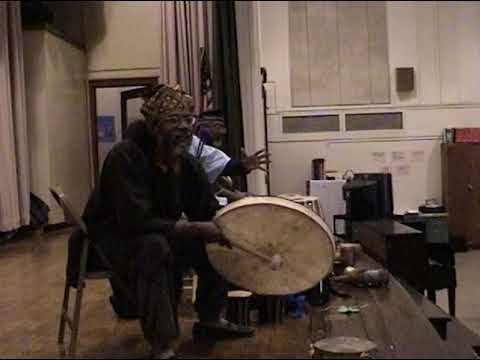In this color photograph, an older African American man with a gray beard and mustache sits on a brown folding chair on a wooden stage. He wears a traditional headdress in shades of brown and yellow, glasses, a black hoodie, and black pants. The man holds a traditional drum with his left hand and a drumstick with a white, rounded end in his right hand. The stage is set up with various instruments, including maracas, bongos, and a piano, suggesting a rehearsal in progress. Behind him, another man in a light blue shirt is partially visible, extending his hand forward in discussion or instruction. The setting appears to be a school auditorium, with white walls and a television, creating an atmosphere of preparation and collaboration.